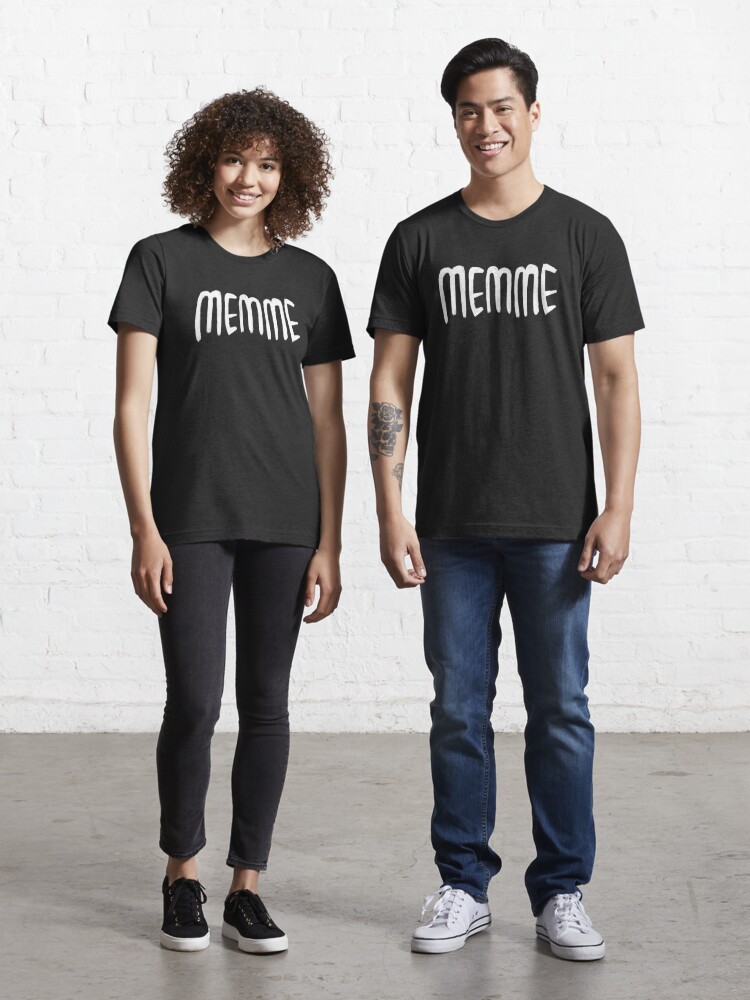Two young models, a man and a woman, stand in an open warehouse area against a white-painted brick wall with a gray concrete floor. Both are dressed in identical black crew neck t-shirts with short sleeves, featuring the word "M-E-M-M-E" in a comic-sans-like white font across the chest, which means "craven" or "cowardly" in German, often referred to as "sissy essential t-shirts." The woman, standing on the left, has curly dark hair, is smiling at the camera, and is dressed in dark blue jeans and black sneakers with white soles. The man, on the right, who has short dark hair and a visible tattoo on his right forearm, complements her with lighter blue jeans and white sneakers. Both models, who appear to be in their early twenties, project a casual and approachable style, making it look like an advertisement setup for these distinctive comic t-shirts.